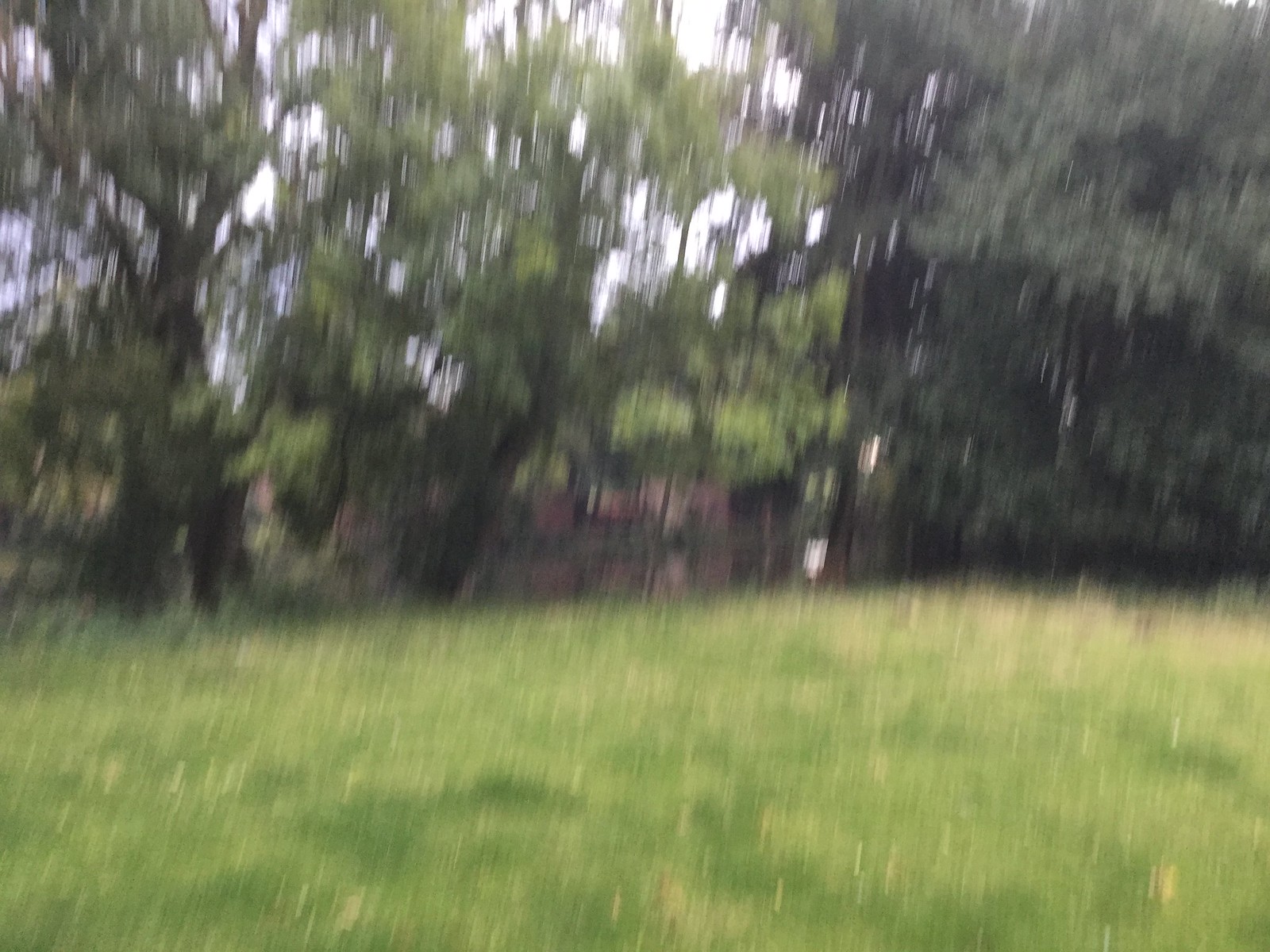In this slightly horizontally rectangular, and excessively blurry exterior photograph captured in natural light, a peaceful scene unfolds. The upper portion of the image, from just below the horizontal center upwards, reveals the silhouettes of several trees. Their leaves vary in shades from very dark green to bright, vivid green, painting the scene with a lush and verdant canopy. Below this, the middle section of the image features what appears to be a small, meandering stream. This stream acts as a divider between the trees above and the area of high grass below. The lower portion of the photo, from just below the stream downwards, showcases tall grasses in various hues of green, creating a rich tapestry of natural textures and colors. Despite the excessive blurriness, the serene beauty of this outdoor setting is palpable, capturing a moment of tranquil harmony within nature.